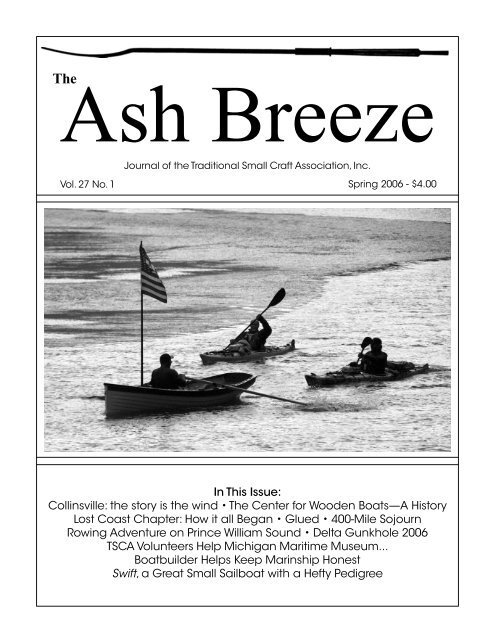The cover of the Spring 2006 issue of *The Ash Breeze*, a black and white journal by the Traditional Small Craft Association, Inc., features a clean, white background with black text. At the very top, a black silhouette of a wooden paddle stretches across the width of the page. Below this, the title "The Ash Breeze" is prominently displayed in large lettering. Directly underneath, in smaller print, is the subtitle "Journal of the Traditional Small Craft Association, Inc." On either side, the details of the issue are noted: in the lower left corner, "Vol. 27, No. 1," and in the lower right, "Spring 2006 - $4." 

Centrally positioned on the cover is a black and white photograph of three men in boats: two in canoes and one in a smaller paddle boat adorned with an American flag. The men and their boats are silhouetted against the background, with hints of a shoreline appearing faintly behind them. The water surrounding the boats seems shallow, with an oar visibly cutting through it.

At the bottom of the cover, a highlighted section reads "In this issue:" and lists various articles, including "Collinsville: The Story is the Wind," "The Center for Wooden Boats: A History," "Lost Coast Chapter: How It All Began," "Glued: 400-Mile Sojourn Rowing Adventure on Prince William Sound," "Delta Gunkhole 2006," "TSCA Volunteers Help Michigan Maritime Museum," "Boat Builder Helps Keep Marine Ship Honest," and "Swift: A Great Small Sailboat with a Hefty Pedigree."